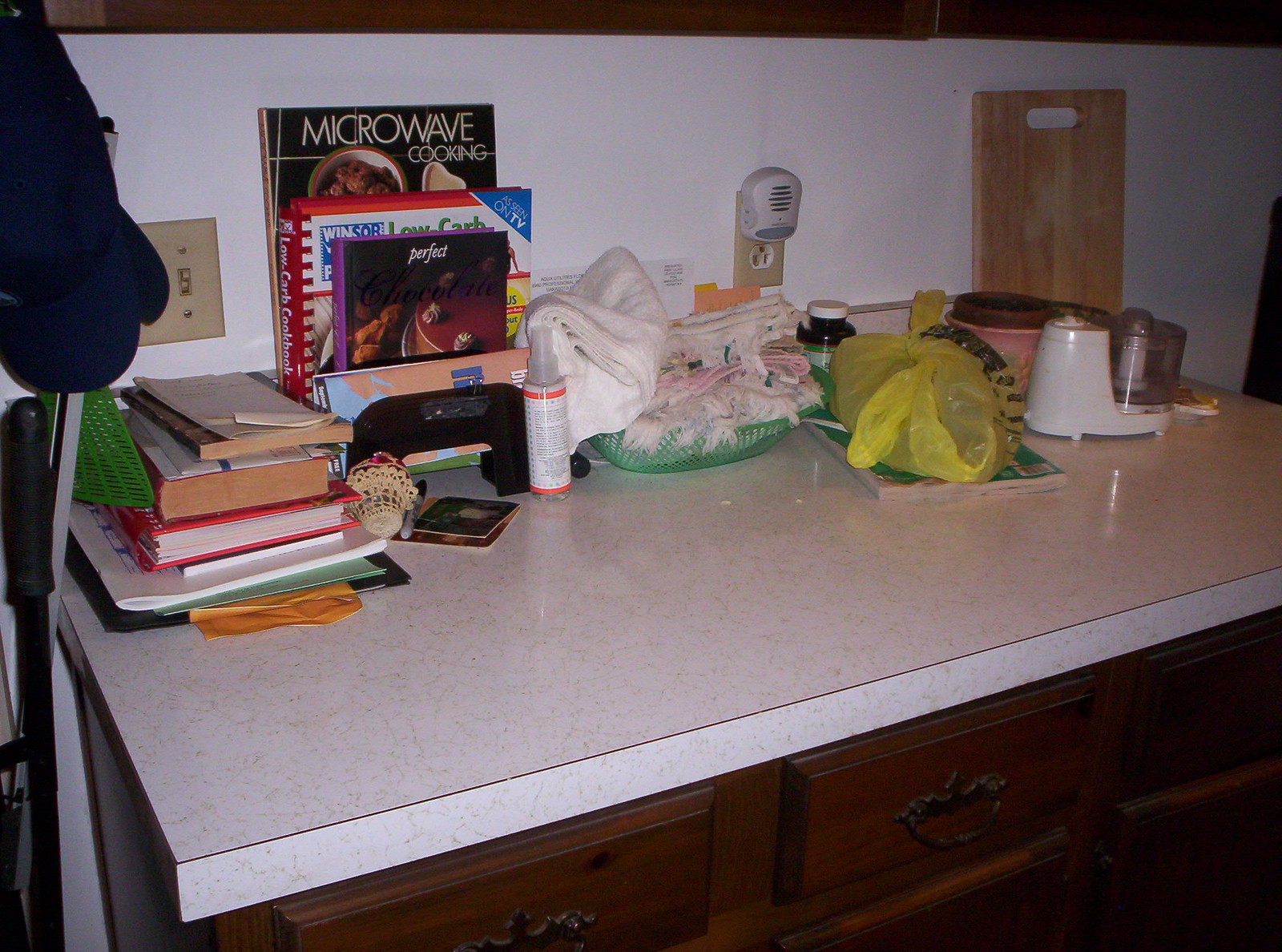The image captures an older Formica countertop with dated cabinetry featuring antique drawer pulls. The countertop is cluttered with various items, primarily books—many of which appear to be cookbooks, including a notable microwave cooking guide. These books are propped up against the wall using a combination of a book holder and a bookend. Among the items on the countertop, there's a noticeable small white food processor positioned in front of a round pink container, which appears to be a pot possibly housing a brown object that might also be used for plants. Adjacent to this scene, a green basket brimming with miscellaneous items is placed, along with a plugged-in scent diffuser.

A white towel lies near a bottle of an unspecified substance, while a yellow plastic bag rests atop a book that resembles a coloring book. The background includes a butcher block cutting board with a handle, leaning against the wall, and an old-fashioned light switch. To the left of the countertop, a black jacket is draped, alongside what appears to be the handle of a broom. This composition creates a nostalgic environment, rich with everyday kitchen essentials and a sense of lived-in history.